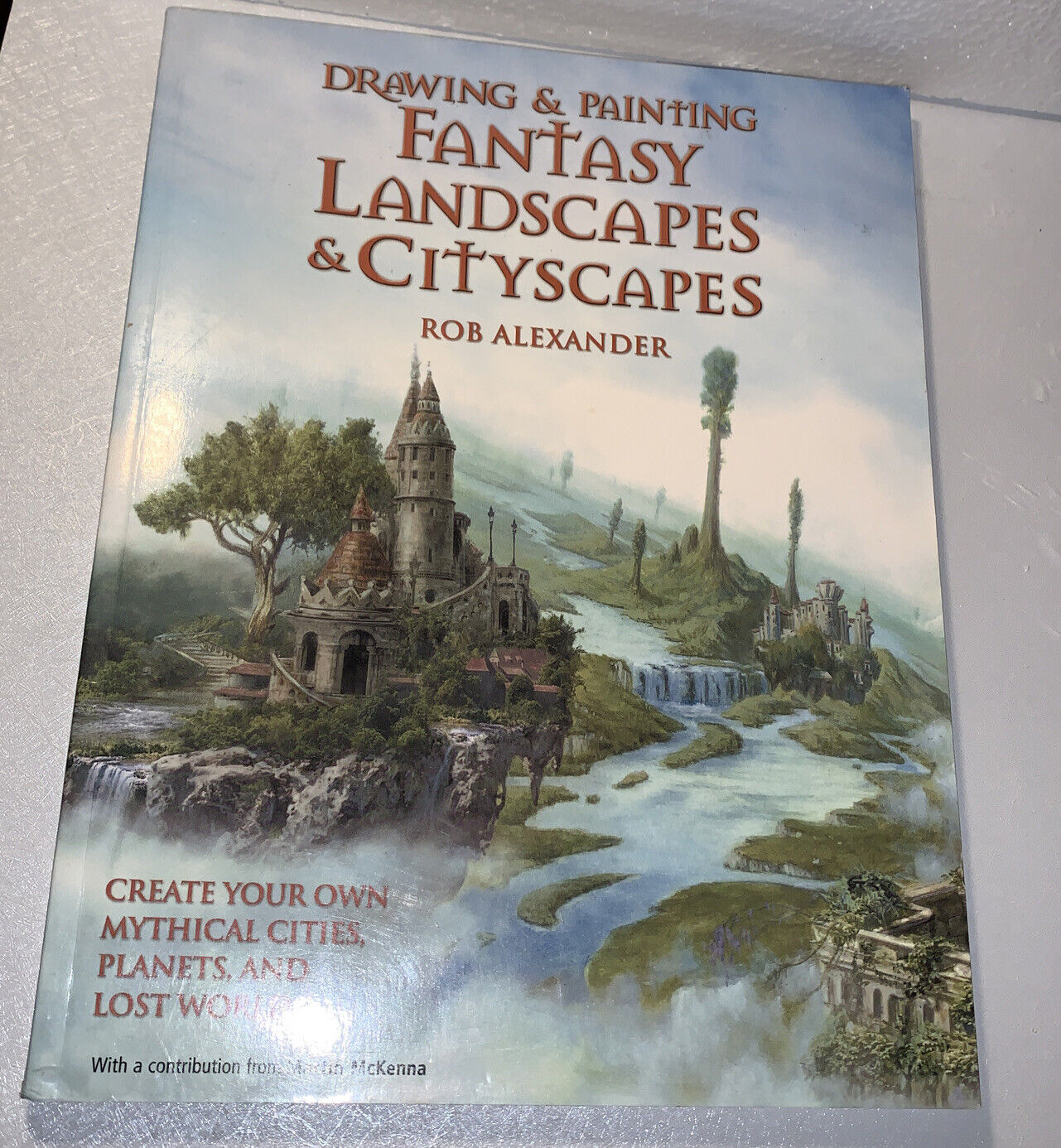The image depicts the cover of a magazine titled "Drawing and Painting Fantasy Landscapes and Cityscapes" by Rob Alexander. Positioned on a white surface, possibly styrofoam, and set against a white wall, the cover showcases a detailed fantasy painting. The central artwork features a dramatic landscape with a majestic waterfall cascading between two rocky, grassy hills. The left side highlights a large castle with spires, spiral staircases, and twisty trees clinging to the rocks. On the opposite hill, which mirrors the first, there is another waterfall and a smaller castle, surrounded by lush foliage. Mist envelops the base of these structures, adding to the mystical atmosphere.

The title, written in a brownish-red, beveled font with a light drop shadow, stands prominently at the top of the cover. The author's name, Rob Alexander, appears smaller under the main title. At the bottom left corner of the cover, a red tagline encourages readers to "create your own mythical cities, planets, and lost worlds" and includes a contribution from Martin McKenna. A glare from the camera flash partially obscures this text, making it difficult to read. This image captures the intricate and enchanting details of the magazine cover, blending elements of fantasy art with practical instructional content.